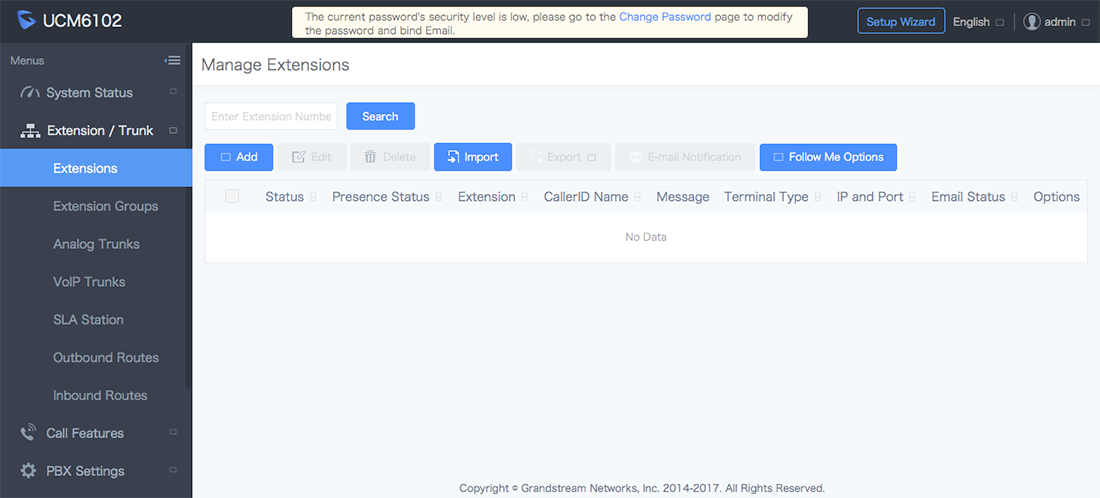This screenshot captures a page from an unidentified website or application, specifically related to Grandstream Networks. At the bottom center in small text, it reads, "Copyright, Grandstream Networks Incorporated, 2014 to 2017, All Rights Reserved." 

In the top left corner, next to a blue logo, the text reads "UCM6102." Central to the top of the page is an important security notice stating, "The current password security level is low. Please go to the change password page to modify the password and bind email." To the right, there is a prominent blue button labeled "Setup Wizard."

The left side of the page features a vertical menu with categories listed from top to bottom as follows: "System Status," "Extension/Trunk," "Call Features," and "PBX Settings." Under the "Extension/Trunk" category, the subcategories are detailed from top to bottom: "Extensions," "Extension Groups," "Analog Trunks," "VoIP Trunks," "SLA Station," "Outbound Routes," and "Inbound Routes."

The "Extensions" subcategory is currently selected. The main section of the page is headed with the title "Manage Extensions."